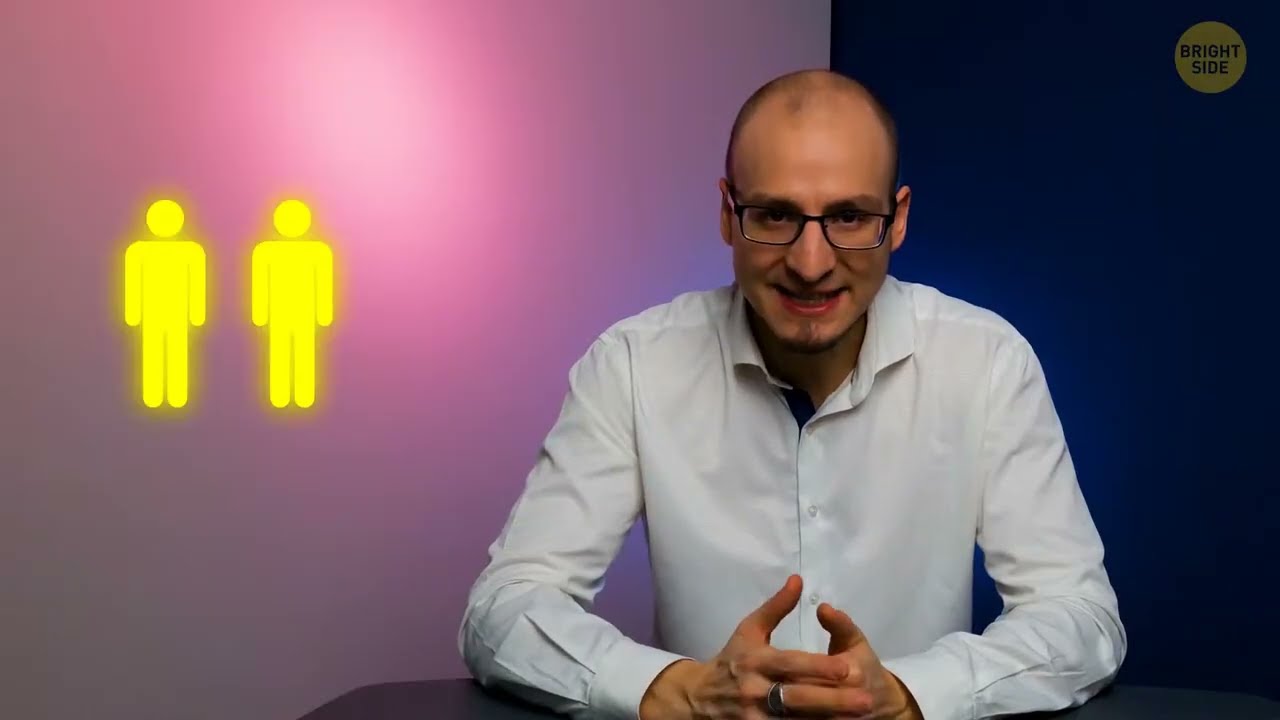In this image, a man with sparse hair, almost bald, is the focal point. He has black-framed glasses, a goatee, and distinctively red lips. His expression is a slight grimace with his mouth partially open. He is seated with his elbows and clasped hands resting on a plain black table, displaying a ring on one finger. He is dressed in a white button-down shirt with some dark coloring near the collar. The background is split horizontally: the left side features a blurred purple wall with two glowing yellow male restroom figures, and the right side is predominantly dark blue. In the upper right, a yellow circle with a translucent text reads "BRIGHT SIDE," suggesting a logo or trademark in the image.